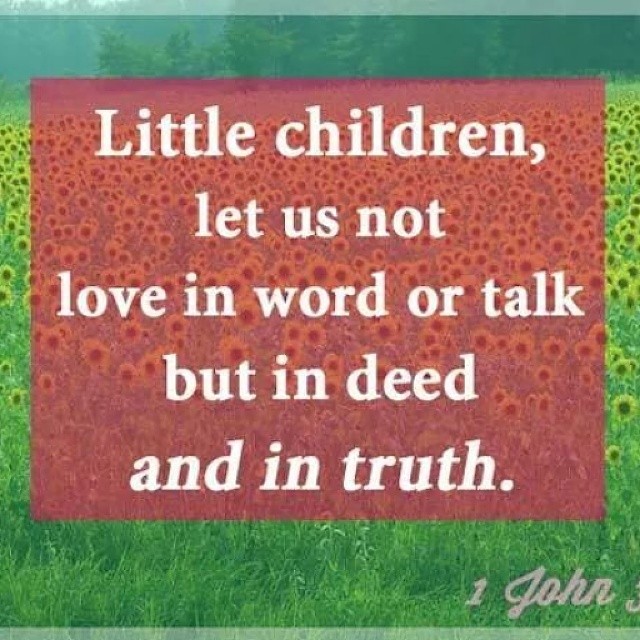The image features a graphic text overlay on a background composed of a field of sunflowers and grass, with taller trees visible in the distance. In the center of the image is a translucent red rectangle containing white text that reads, "Little children, let us not love in word or talk, but in deed and in truth." In the bottom right-hand corner, there is gray text that partially reads, "One John," suggesting a quote from the New Testament. The background behind the text is somewhat blurred, as if seen through glass, creating an impressionistic effect. The majority of the sunflowers are concentrated in the upper third of the image.